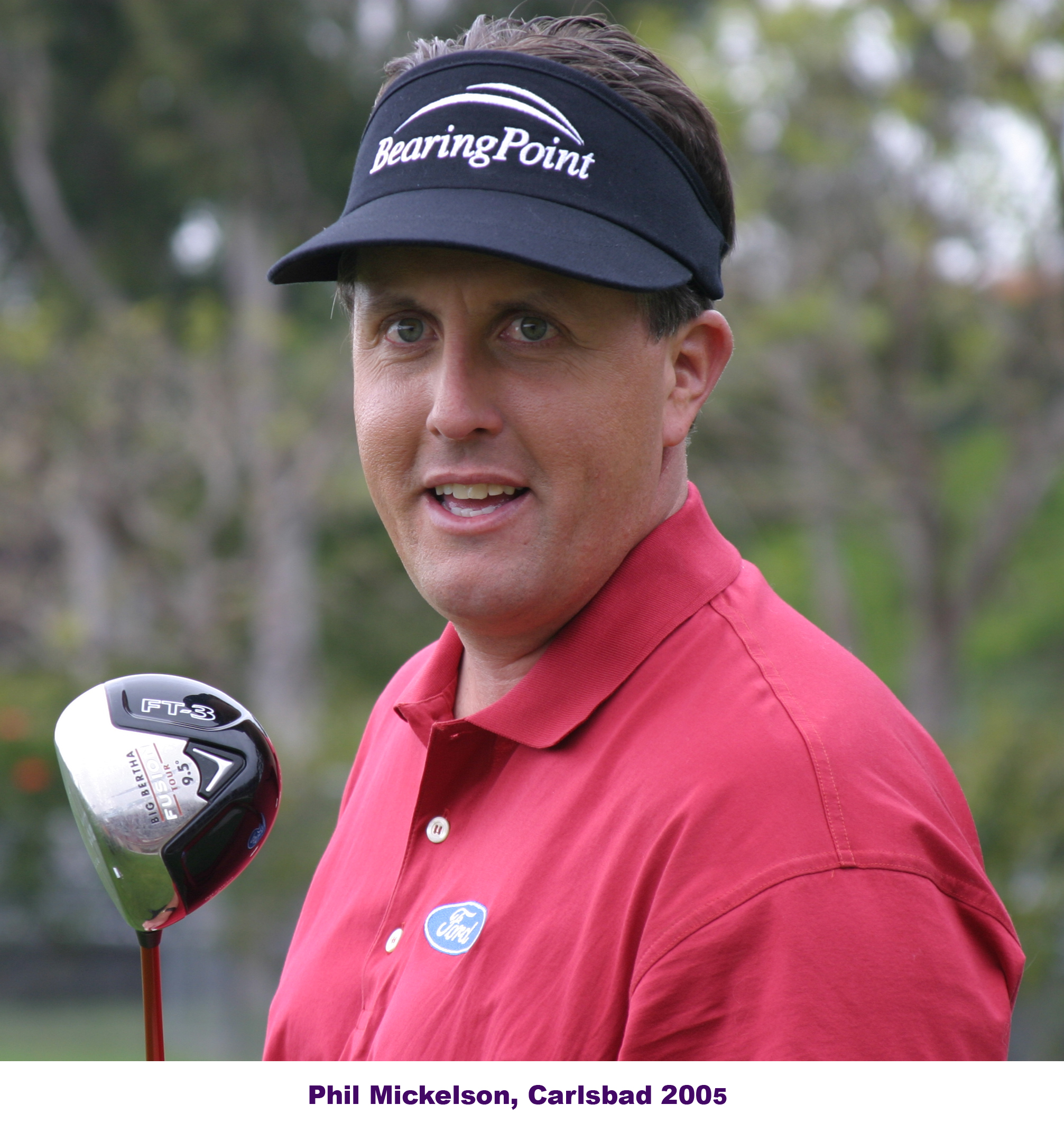This close-up photograph, taken outdoors on a sunny day, depicts the celebrated golfer Phil Mickelson. He is captured wearing a red button-up collared shirt adorned with a Ford patch on the right side of his chest. Mickelson is sporting a black golf visor with "Bearing Point" written in white text. His light green or light blue eyes gaze towards the camera, and he is seen holding a black and silver golf club with the marking "9.5" on its head. The background is softly blurred, revealing a landscape of trees, branches, and trunks. At the very bottom of the image, a white strip of text in light purple states, "Phil Mickelson, Carlsbad, 2005," with the digit '5' notably smaller than the other characters.